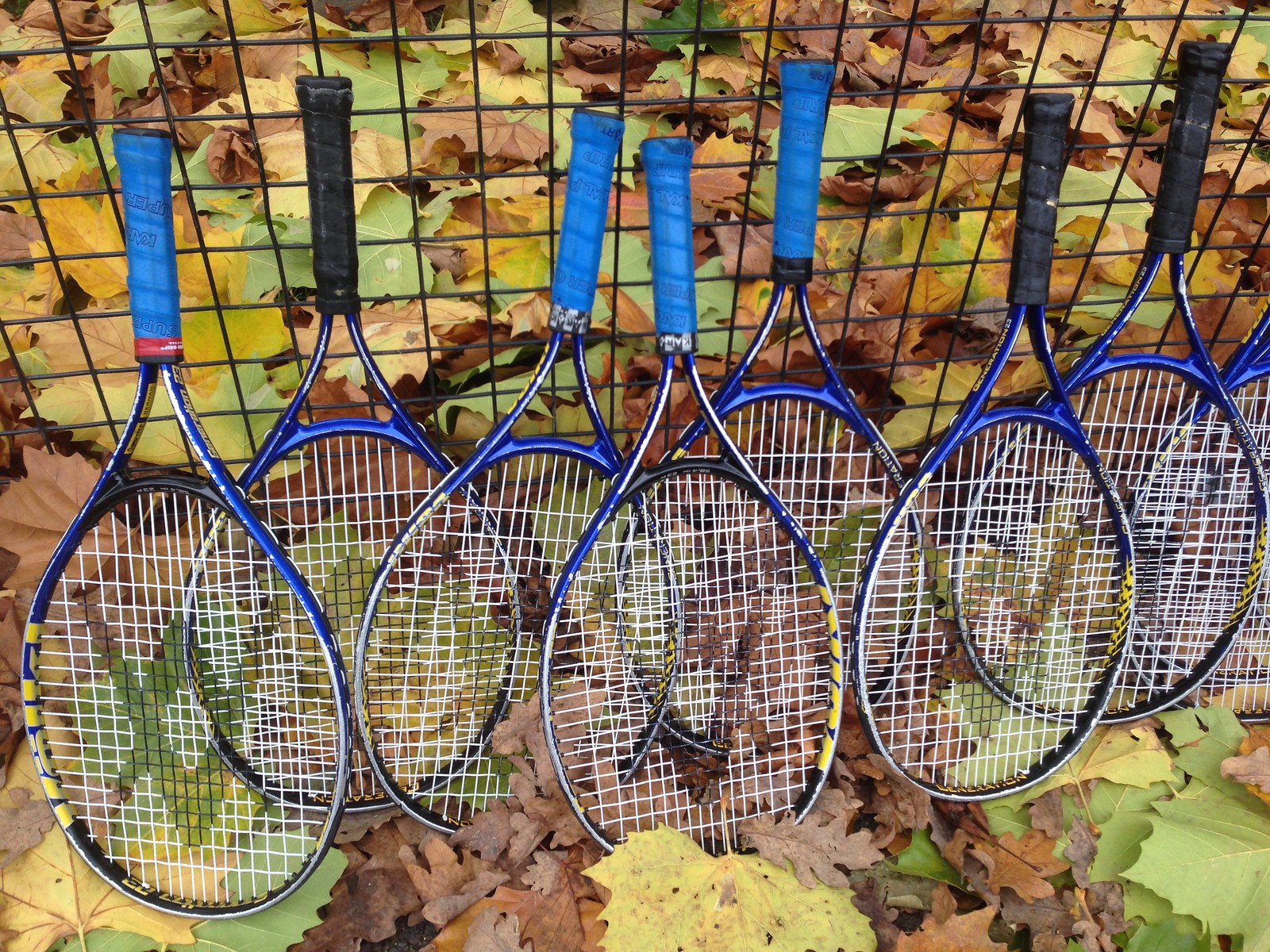This outdoor photograph, taken in the fall, features seven full tennis rackets and part of an eighth one, all propped up against a black, metal grid fence with square patterns. The vibrant autumn background is filled with leaves in shades of light green, yellow, brown, and tan, carpeting both the ground and the area behind the fence. The tennis rackets, aligned in a horizontal row with their handles pointing up, consist of four with blue handles and three with black handles. The rackets have blue frames with some white striping and yellow markings, and their netting features a distinctive diamond pattern. This detailed scene captures a serene autumn setting, possibly near a tennis court not visible in the image.